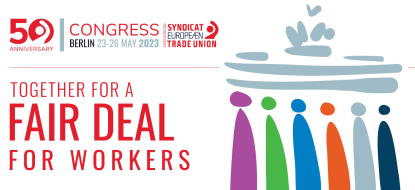The image is a detailed print advertisement celebrating the 50th anniversary of the Syndicate European Trade Union Congress, scheduled to be held in Berlin from May 23 to 26, 2023. The design features a clean, white background, blending seamlessly with the surroundings, and is in landscape orientation, wider than it is tall. At the top left corner, prominent red text declares "50th Anniversary," with the zero stylized as an arm extending upward from its center. Directly beneath and to the right, it continues with "Congress" in red, "Berlin" in black, and "23-26 May 2023" in light blue.

Further to the right, the words "Syndicate" in red, "European" in blue, and "Trade Union" in red are followed by a small image of a human figure waving their arm. Below this central header, a horizontal gray line separates the top from the bottom part of the advertisement. The bottom left corner highlights a bold, red slogan: "Together for a Fair Deal for Workers."

The right half of the image features a visually striking representation of a fountain at the top and six stylized figures beneath, each consisting of a dot (head) and a vertical bar (body). These figures are colored purple, green, blue, orange, gray, and black. The overall design emphasizes the unity and diversity of the trade union through these vibrant, colorful elements.